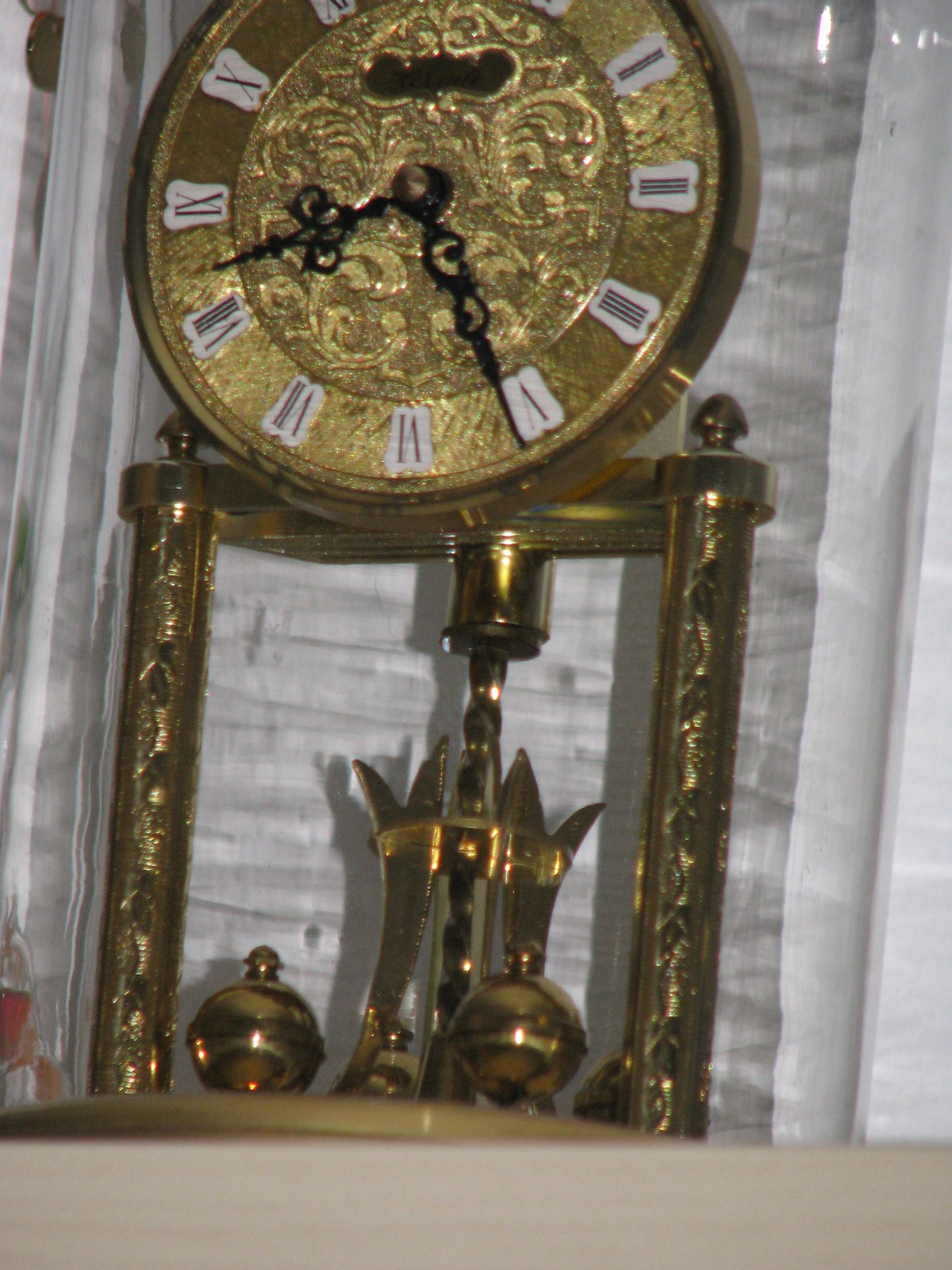A vintage clock with a golden-hued face is enclosed within a glass dome. The time displayed on the clock is 8:26. This model, popular in the 1980s and 1990s, features an ornate design with intricate detailing. The clock stands on three elegant legs and is powered by a AA battery inserted at the back. Below the clock face, three spinning balls add a dynamic element to its classic charm. This nostalgic piece is reminiscent of a bygone era, evoking fond memories for many who owned such a clock in their homes.